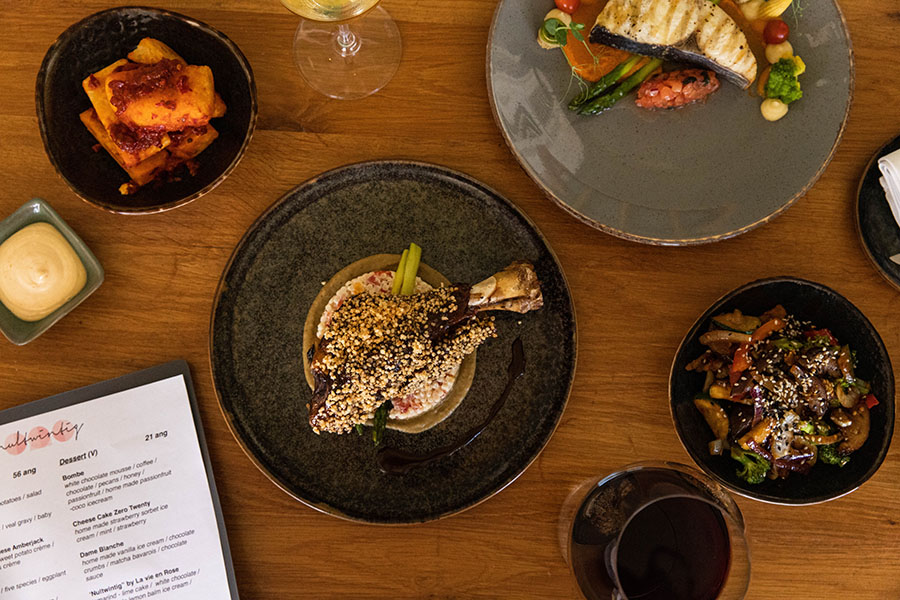In this photograph taken at a fancy restaurant, a pristine wooden table is artfully arranged with a variety of dishes and drinks. On the bottom right-hand corner, a stylishly designed menu prominently displays dessert options. The table setting includes a sophisticated spread: in the top left corner, there is a square ceramic dish, possibly with a custard-like dessert. A small bowl of dipping sauce, likely balsamic vinegar, accompanies a piece of bread positioned in the top right-hand corner, hinting at a classic balsamic and olive oil pairing.

Central to the arrangement are several elegantly presented main courses. A gray plate holds a grilled white fish paired with colorful, grilled vegetables. Nearby, another dish features what looks like a lamb shank encrusted with nuts, providing a rich, textured contrast. There is also a dish with vegetables garnished with sesame seeds, possibly accompanied by soy sauce, adding an Asian-inspired flair. A hint of a wine glass with what appears to be white wine can be seen at the top of the image, completing the sophisticated dining experience. Each plate is meticulously plated, reflecting the restaurant's exquisite attention to detail and culinary craftsmanship.